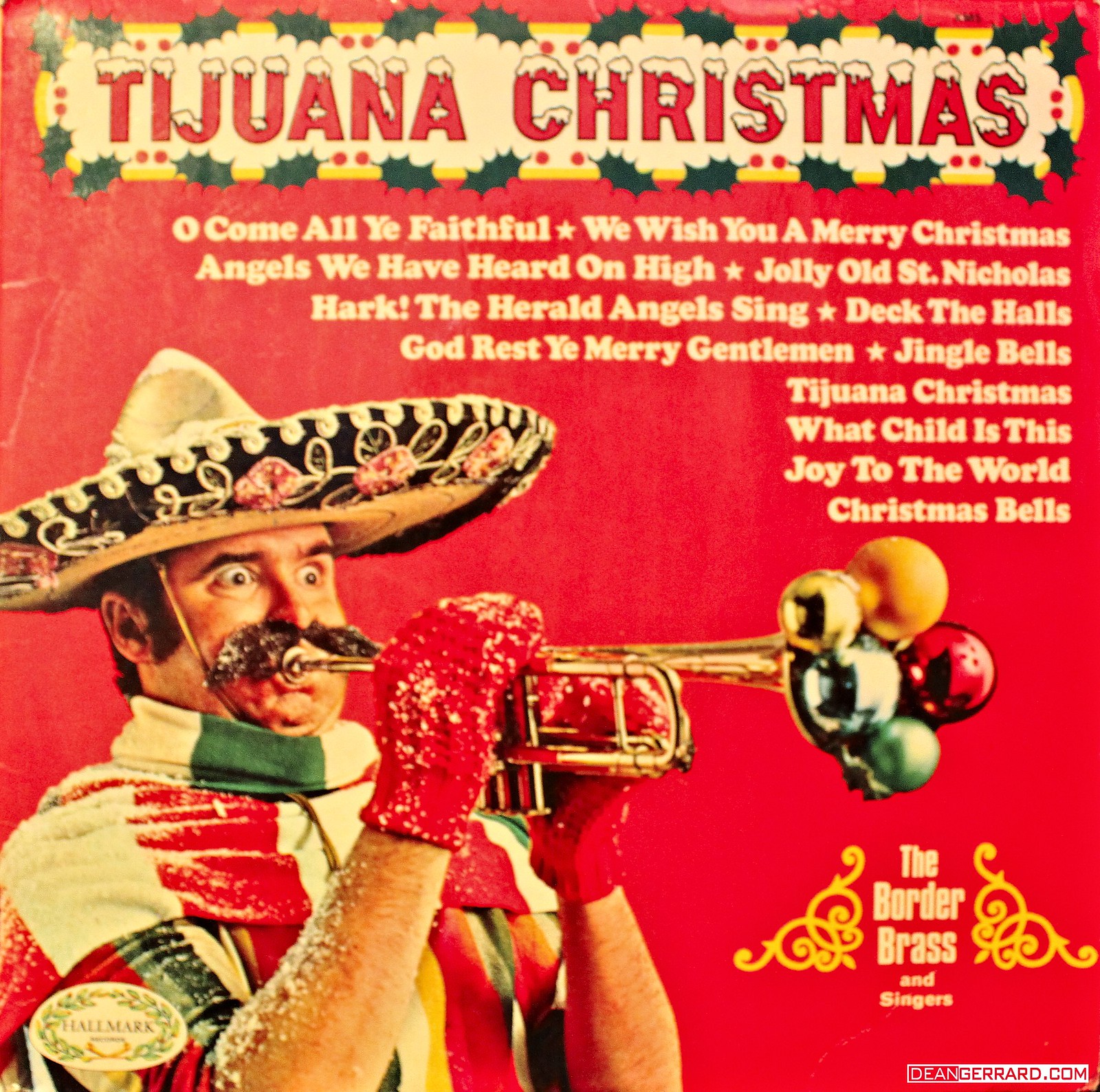The image is an album cover with a festive Mexican Christmas theme. At the top, against a white banner adorned with mistletoe leaves, the title "Tijuana Christmas" is prominently displayed in red letters, each topped with a dusting of snow. Surrounding the banner is a border embellished with holly leaves and a yellow line. Below the title, in white text, is a list of Christmas tracks including "O Come All Ye Faithful," "We Wish You a Merry Christmas," "Angels We Have Heard on High," "Jolly Old St. Nicholas," "Hark the Herald Angels Sing," "Deck the Halls," "God Rest Ye Merry Gentlemen," "Jingle Bells," "Tijuana Christmas," "What Child is This," "Joy to the World," and "Christmas Bells." 

In the center left of the cover, there is an image of a Hispanic man dressed festively in a red, white, and green poncho, with a matching scarf, and a sombrero. He has a bushy mustache and an exaggerated, leafy beard. The man is playing a trumpet filled with Christmas ornaments and appears to have gloves and traces of snow on him. At the bottom right, the text reads "The Border Brass and Singers," associated with DeanGirard.com. The background is predominantly red with some gold highlights, completing the vibrant holiday theme.